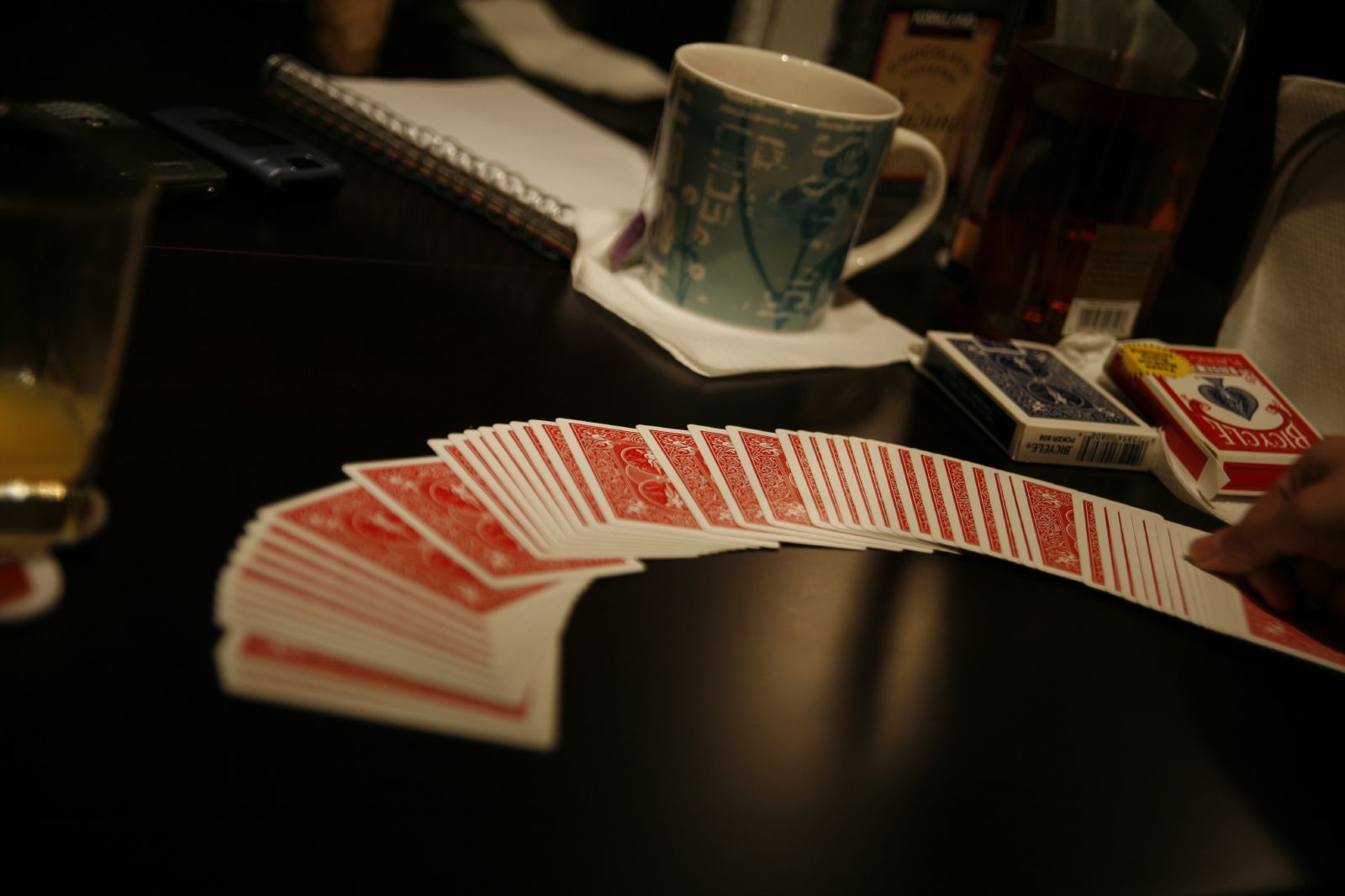A mesmerizing photograph captures a red Bicycle playing card deck meticulously fanned out across a table, resembling a graceful Nike swoosh, thickest on the left and tapering to the right. The scene is animated by a right hand gently resting on the cards, suggesting a moment mid-card trick. Just behind this visual flourish, the red box that the cards came from sits prominently, flanked by a similar blue Bicycle card box. Adding an element of realism, a blue and white ceramic mug placed on a paper napkin sits to the left of the card boxes. In the background, an open spiral-bound notebook lies open, hinting at notes or doodles possibly related to the card magic at hand. Further back, a couple of alcohol bottles make a subtle appearance. One bottle shows a visible barcode but remains somewhat mysterious with a lighter Coca-Cola hue to its liquid, while the other is unmistakably adorned with the Kirkland logo from Costco, revealing an unexpected foray into the world of spirits. The entire ensemble offers a fascinating glimpse into an eclectic mix of leisure and magic.